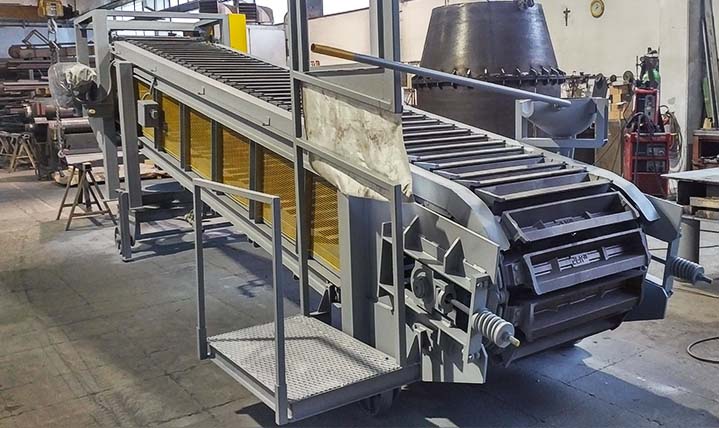The photograph captures a detailed view of a stationary, industrial conveyor belt located in a factory or warehouse setting. The conveyor belt, angled at around 45 degrees, features a top layer of grey plastic bins. Its underside is highlighted by a yellow component, possibly a net filter or bins, which stands out against the otherwise grey machinery. The scene includes a concrete floor and various pieces of equipment surrounding the conveyor belt. Towards the right, there is a red tool chest, while off to the left, some planks of wood are visible. In the background, a wall adorned with a clock and a cross is partially seen, along with several windows. Additionally, there are three metal workhorses under the conveyor belt, further emphasizing the industrial nature of the environment.